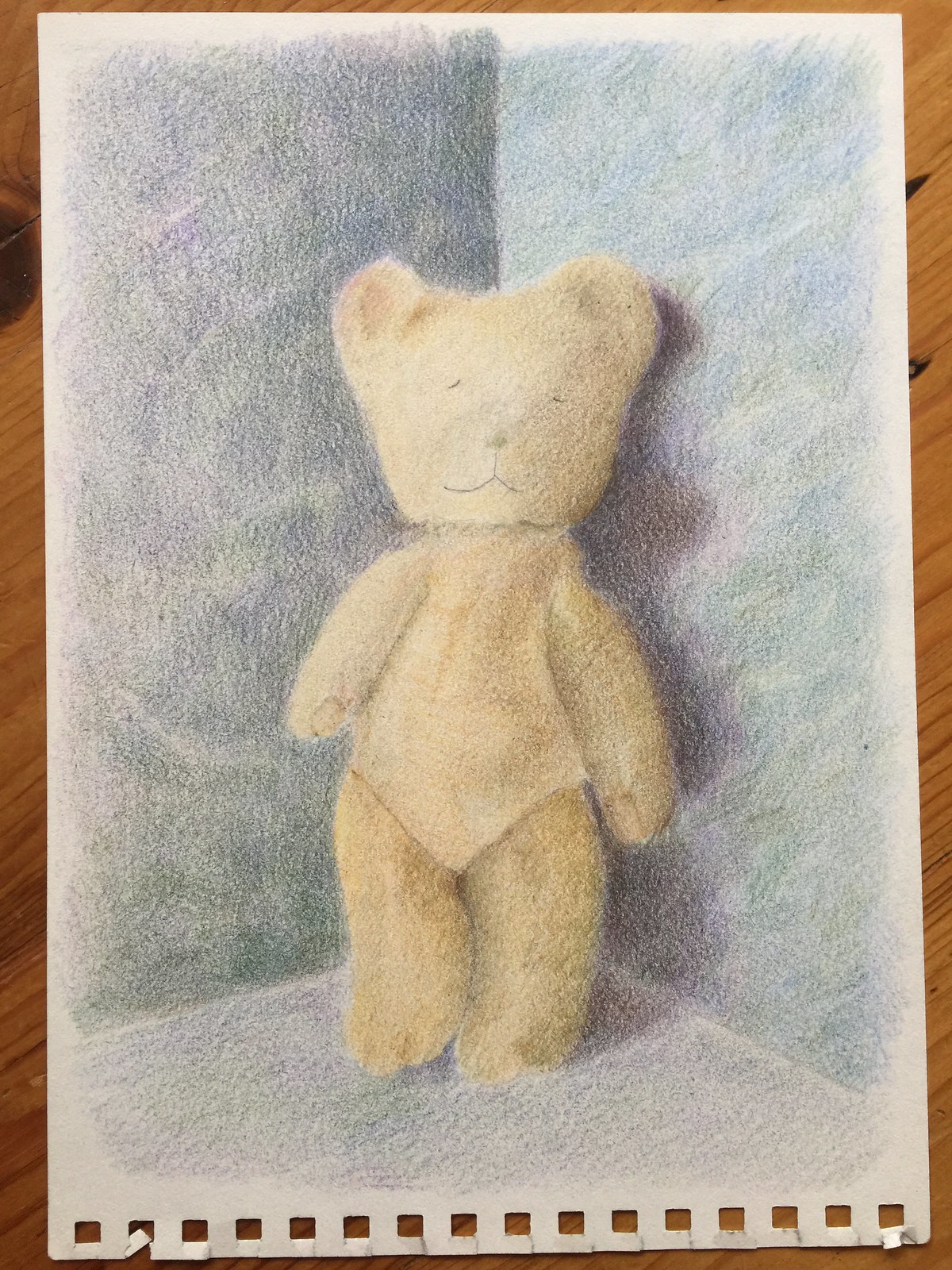This detailed photograph showcases an art piece meticulously crafted on sketchbook paper, which has been torn from its original spiral-bound book, evidenced by the jagged edges visible at the bottom. The sheet rests on a textured wooden table, adding a rustic backdrop to the artwork. The drawing, likely rendered with colored pencils, depicts a serene scene of a brown teddy bear doll leaning against a corner of a room. The teddy bear is portrayed with closed eyes and a gentle, contented smile, capturing a moment of peaceful repose. Its positioning in the corner creates a shadow that falls both on the ground and against the adjacent walls, enhancing the depth and realism of the composition.